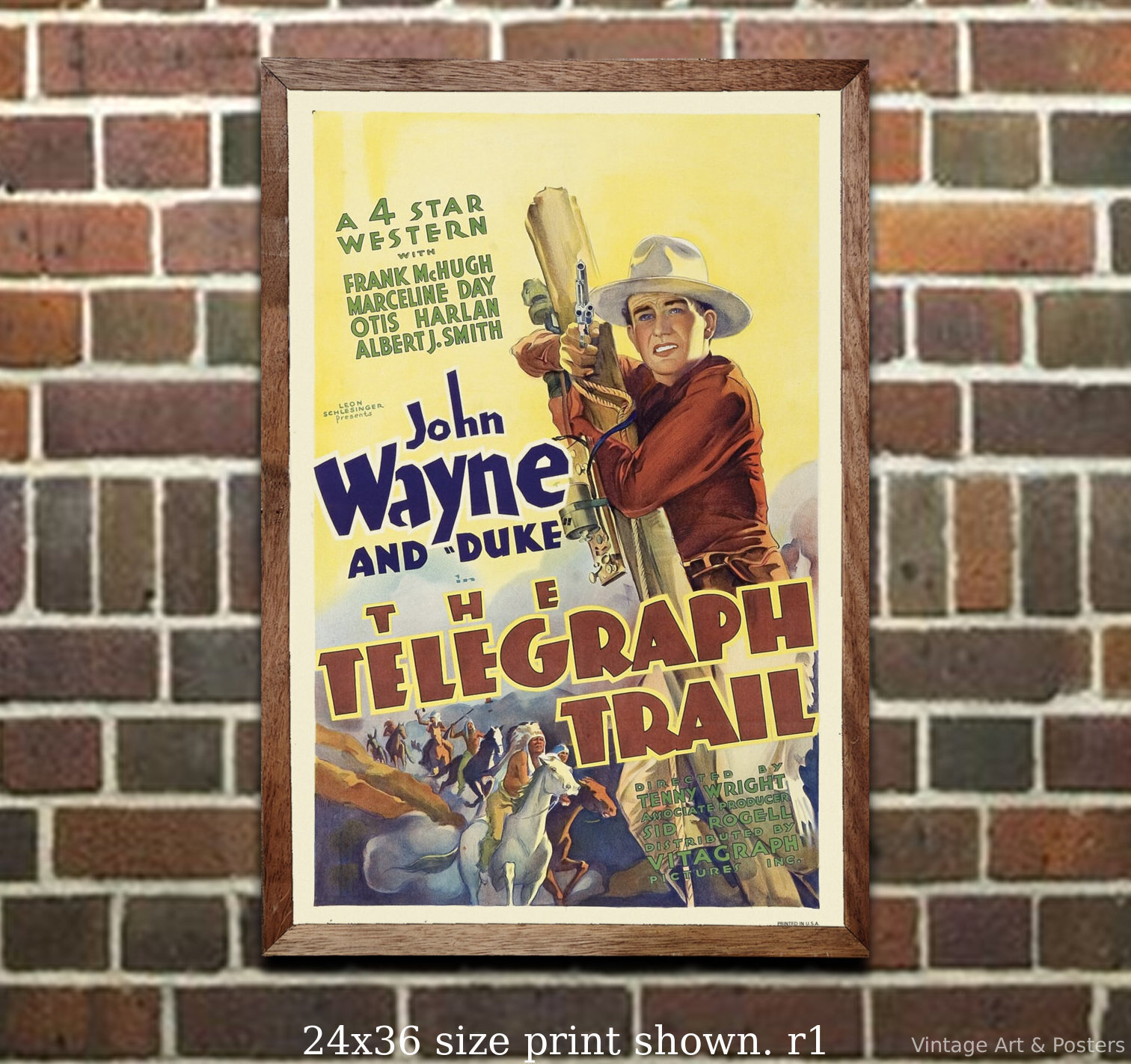On a rustic brick wall, there's a prominently displayed vintage movie poster, framed in natural wood, measuring 24 by 36 inches. This poster advertises a film titled "The Telegraph Trail," starring John Wayne. Above the main image, it boasts "A Four-Star Western" and lists co-stars including Frank McHugh, Marceline Day, Otis Harlan, and Albert J. Smith. The type runs diagonally from the top left-hand corner to the bottom right. Featured at the center is John Wayne, dressed in a red shirt and a large white cowboy hat, gripping a pole with one hand and aiming a gun directly at the viewer with the other. Below him, a vivid scene depicts Native Americans on horses in pursuit. The text at the bottom of the poster reads, "24 by 36 size print shown, R1, Vintage Prints and Posters," indicating that this classic piece of movie memorabilia is available for purchase.